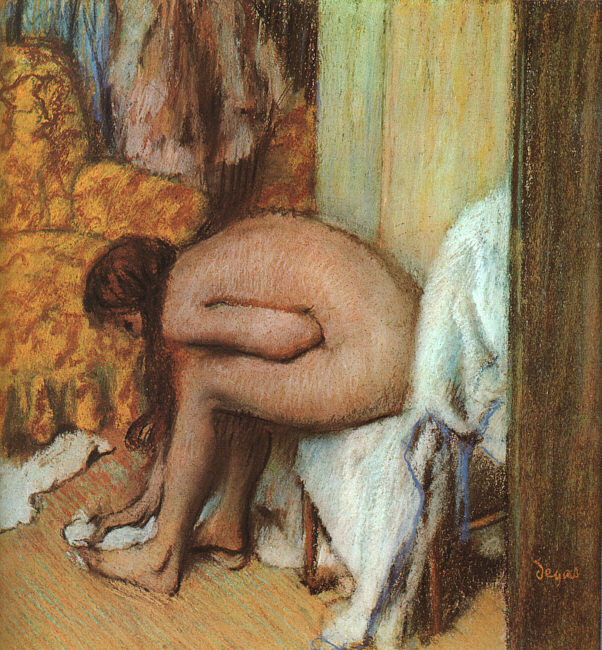This image is a detailed painting by Edgar Degas, done in acrylic. It depicts a young naked woman of Caucasian descent seated on a chair, which is covered with a white dress adorned with a blue ribbon. The woman, who has long, reddish-brown hair cascading over her left shoulder to the ground, is bent over and wiping her foot with a white cloth. Her posture allows the ridgelines of her spine to be visible. The setting includes an orange armchair on the left with a yellow chair cover marked by a red floral pattern. The background of the room features walls in green and yellow tones with a blue doorframe. Along the vertical wooden beam on the right are elements of brown and green hues on the floor, tying the composition together. The artist's signature, "Degas," is noticeable in orange at the bottom right of the painting.